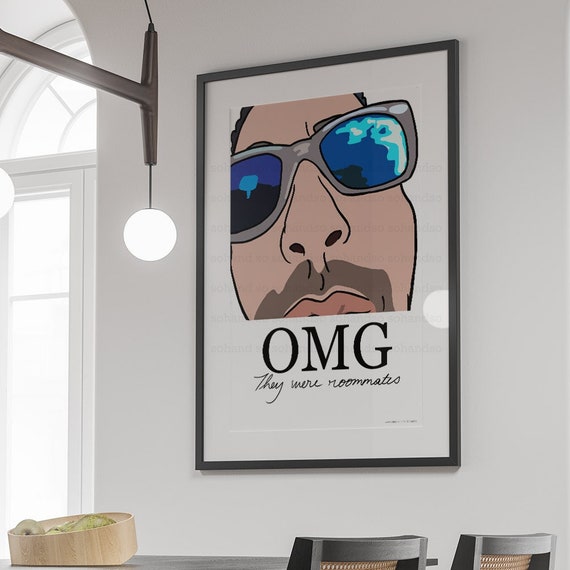The image depicts a warmly lit home interior with a focal point of a striking framed artwork. The space features a large white wall adorned with a cartoon drawing of a man with tan skin, brown goatee or mustache, and vibrant blue-lensed sunglasses that pop against the minimalist background. Beneath the man's face, large bold text exclaims "OMG" with cursive writing below reading "they were roommates." To the left of this artwork, a large arched window bathes the room in natural light, enhanced by a hanging chandelier with glowing spherical bulbs. Complementing the scene, a dark wooden kitchen table is partially visible in the foreground, accompanied by wicker-backed chairs. A light-colored wooden bowl with indistinct contents decorates the table, adding to the cozy and eclectic ambiance.